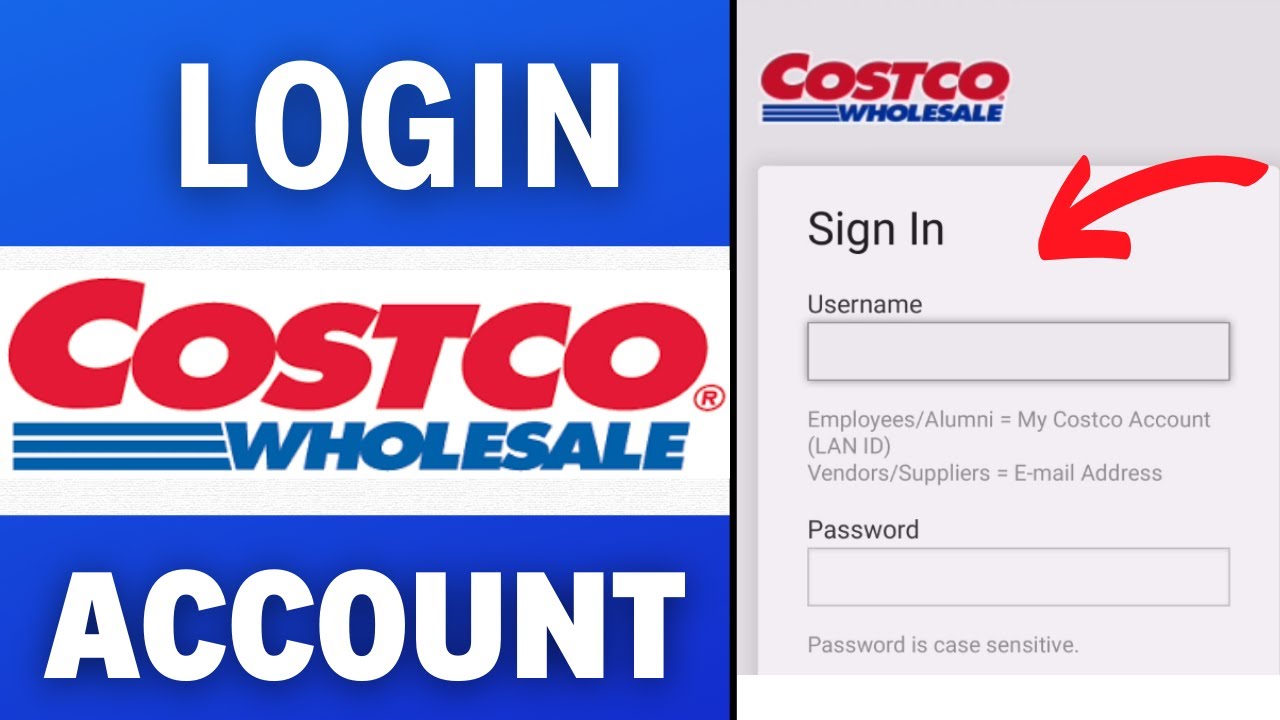The image captured is from a login section for Costco Wholesale. The left side of the image prominently features the word "LOGIN" at the top in white, all capital letters, set against a royal blue rectangle. Below this, the text "Costco Wholesale" is displayed, with "Costco" appearing in red alongside a registered trademark symbol (®) in a red circle. Beneath "Costco," the words "wholesale" and three preceding lines are shown in a navy-blue color. At the bottom, another royal blue rectangle contains the word "ACCOUNT" in white, all capital letters.

On the right side of the image is another emblem that reads "Costco Wholesale," mirroring the brand's characteristic colors and design. Positioned at the top of this section is the "Sign In" area. Here, there is a blank rectangle intended for entering the username, accompanied by the guidance text: "Employees / Alumni = My Costco Account" and "LAN ID Vendor Suppliers = Email Address." Below this is an empty password box labeled "Password is case sensitive." A red arrow points directly to the username field, guiding users on where to begin the sign-in process.